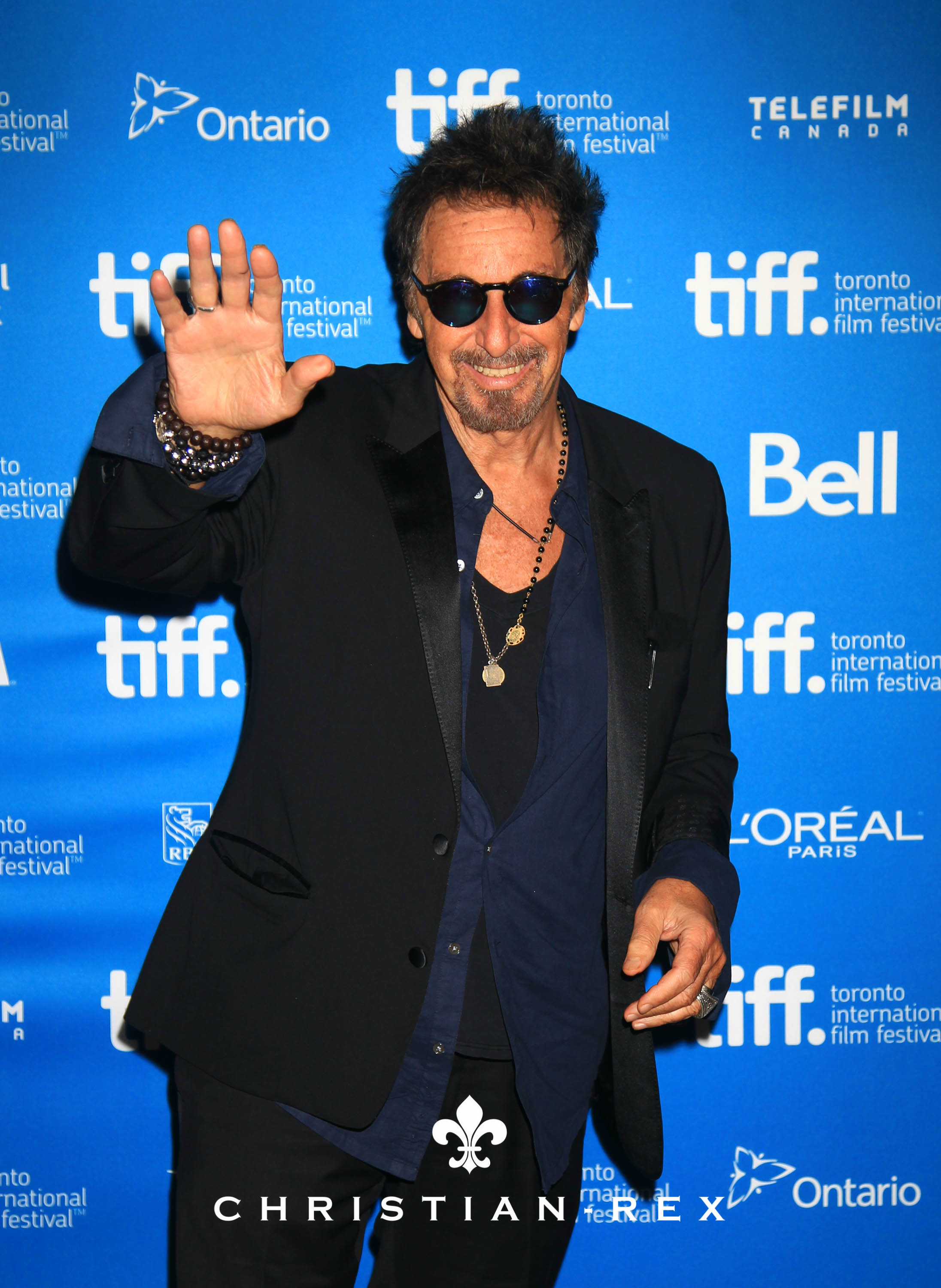A man is posing and waving in front of a blue wall adorned with repeating white logos for Ontario, TIFF (Toronto International Film Festival), Telefilm Canada, Bell, and L'Oreal Paris, suggesting a celebrity event setting. The man is visible from his upper thighs to the top of his head, exuding a stylish appearance. He is wearing black pants and a coordinated black ensemble consisting of a business coat, an undershirt, and a blue button-up shirt with only one button fastened in the center. His accessories include multiple bead bracelets on his raised hand, rings on both hands, necklaces, and black sunglasses. He sports a goatee with a mustache and has full black hair, completing his sophisticated look.